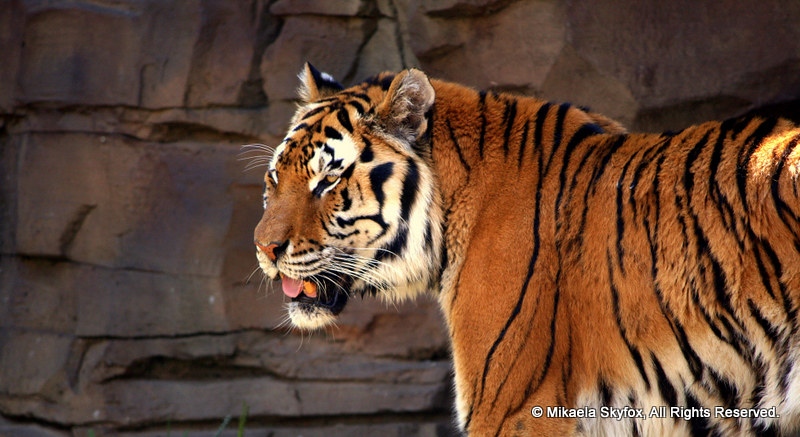In this close-up nature photograph, a striking tiger is the focal point, depicted with meticulous detail. Positioned in the lower right corner of a horizontally oriented frame, the tiger stands side-on, head raised towards the center of the image, looking left. Its body is rendered in vibrant stripes of orange and black, with white fur accentuating its face and areas around its eyes. The tiger's mouth is slightly open, revealing a pink tongue. The background comprises a rocky wall, emphasizing the outdoor setting, likely taken in daylight within a zoo environment. A few blades of grass are visible in the lower left corner. In the bottom right corner, the image bears the watermark "copyright Michaela Skyfox, all rights reserved" in white lettering. The dominant colors are orange, brown, black, white, gray, and pink.